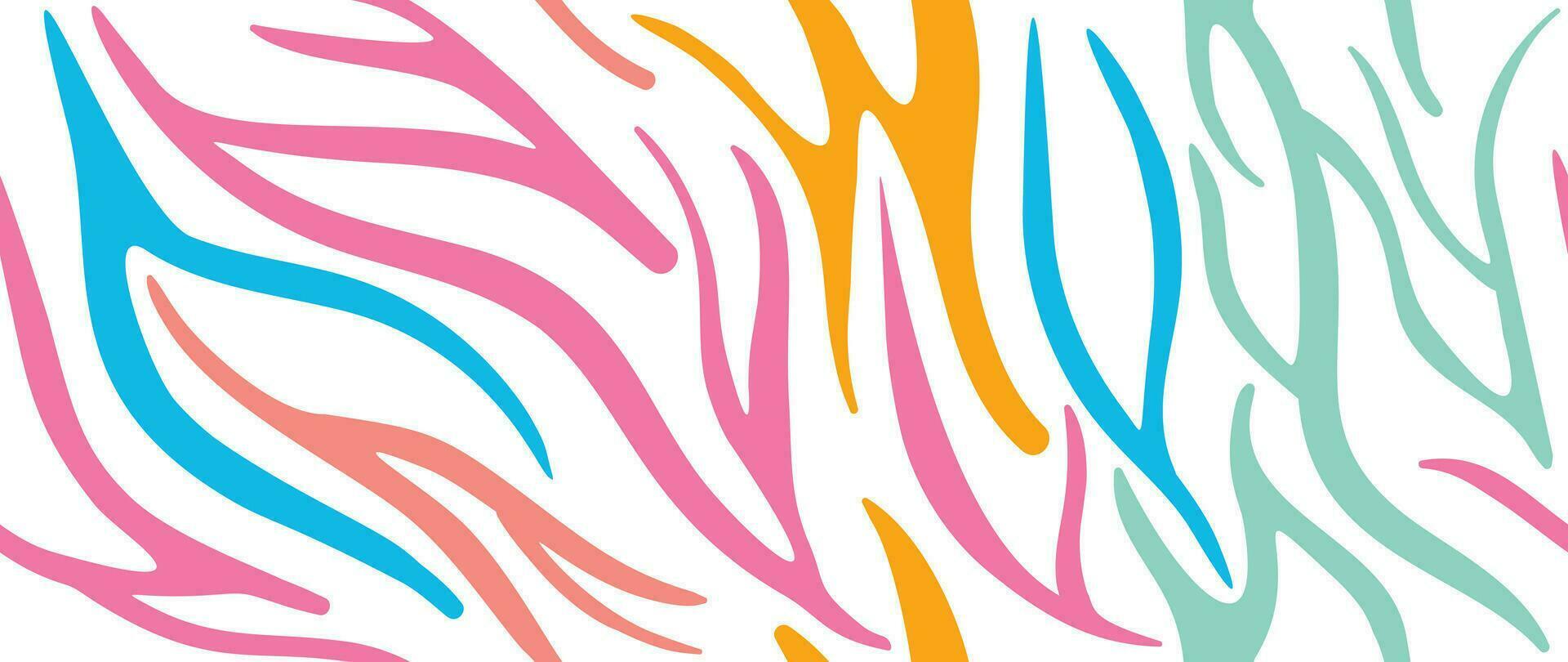This vibrant artwork features an abstract composition reminiscent of zebra stripes, set against a pristine white background. The wide, rectangular piece showcases undulating waves of color that flow from the bottom left to the top right, creating a dynamic sense of motion. Prominent hues include light pink, medium blue, salmon coral, orange, and teal green. The colorful patterns alternate and swirl across the canvas, overlapping and intertwining in a mesmerizing dance. Despite its abstract form, the artwork evokes the rhythmic and organic patterns found in nature, blending elements of both flame-like waves and zebra-like stripes. The combination of bright, varied colors against the white backdrop makes the piece both striking and beautiful, capturing a sense of continuous movement and energy.